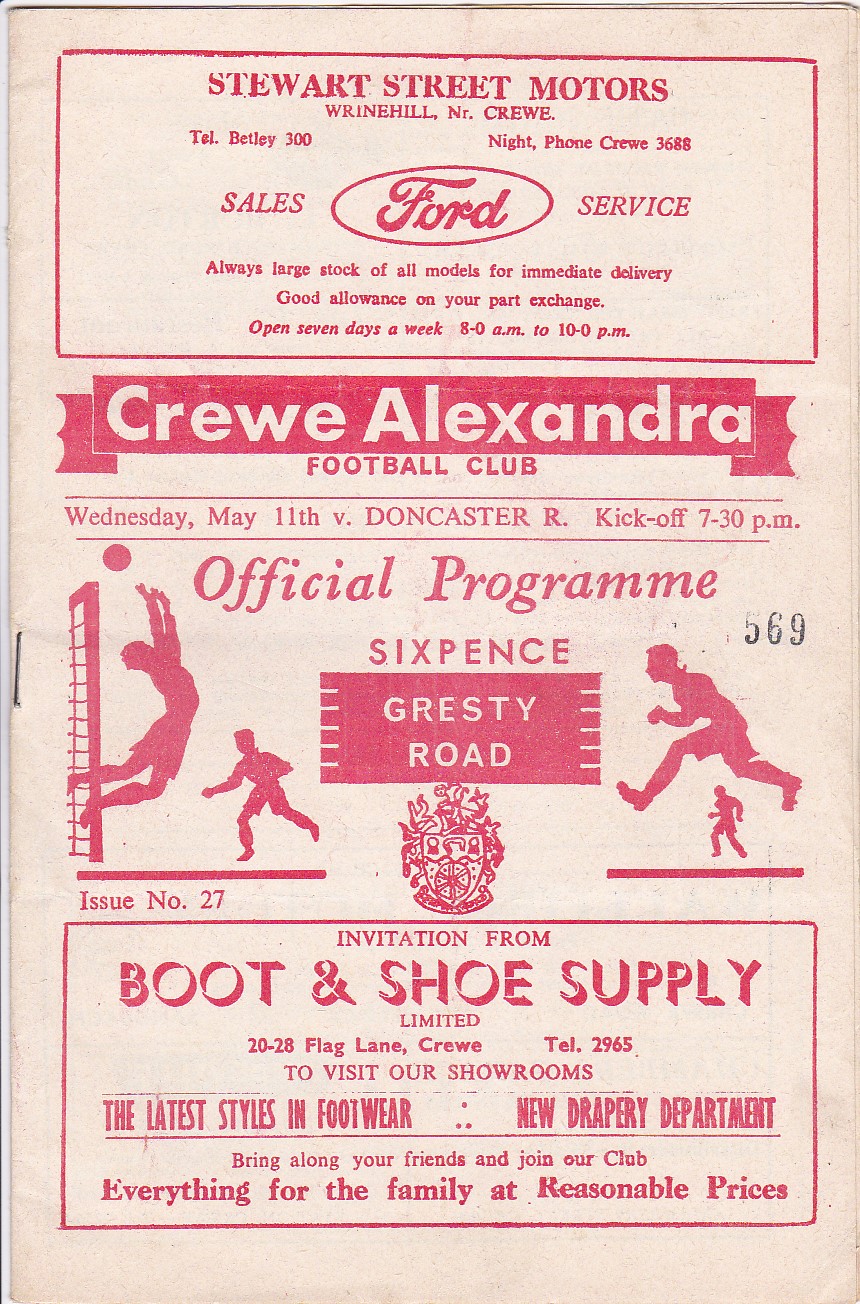The cover of this vintage sports program for Crew Alexandra Football Club features a prominent advertisement at the very top from Stewart Street Motors, a Ford dealership, characterized by its all-white background with red lettering, promoting large stock of all Ford models available and open seven days a week. Below the advertisement, the cover displays the name Crew Alexandra Football Club in bold red text. The program details a match scheduled for Wednesday, May 11th against Doncaster, with kickoff at 7:30 p.m., and mentions that the issue was priced at Sixpence. Central to the cover are red-inked sketches of soccer players framing a flag with the text "Grizzly Road." At the bottom, another red banner advertises Boot and Shoe Supply Limited, inviting readers to explore their latest footwear styles and new drapery department, catering to the entire family at reasonable prices. The entire page utilizes a red and white color scheme, giving it a classic, aged look.